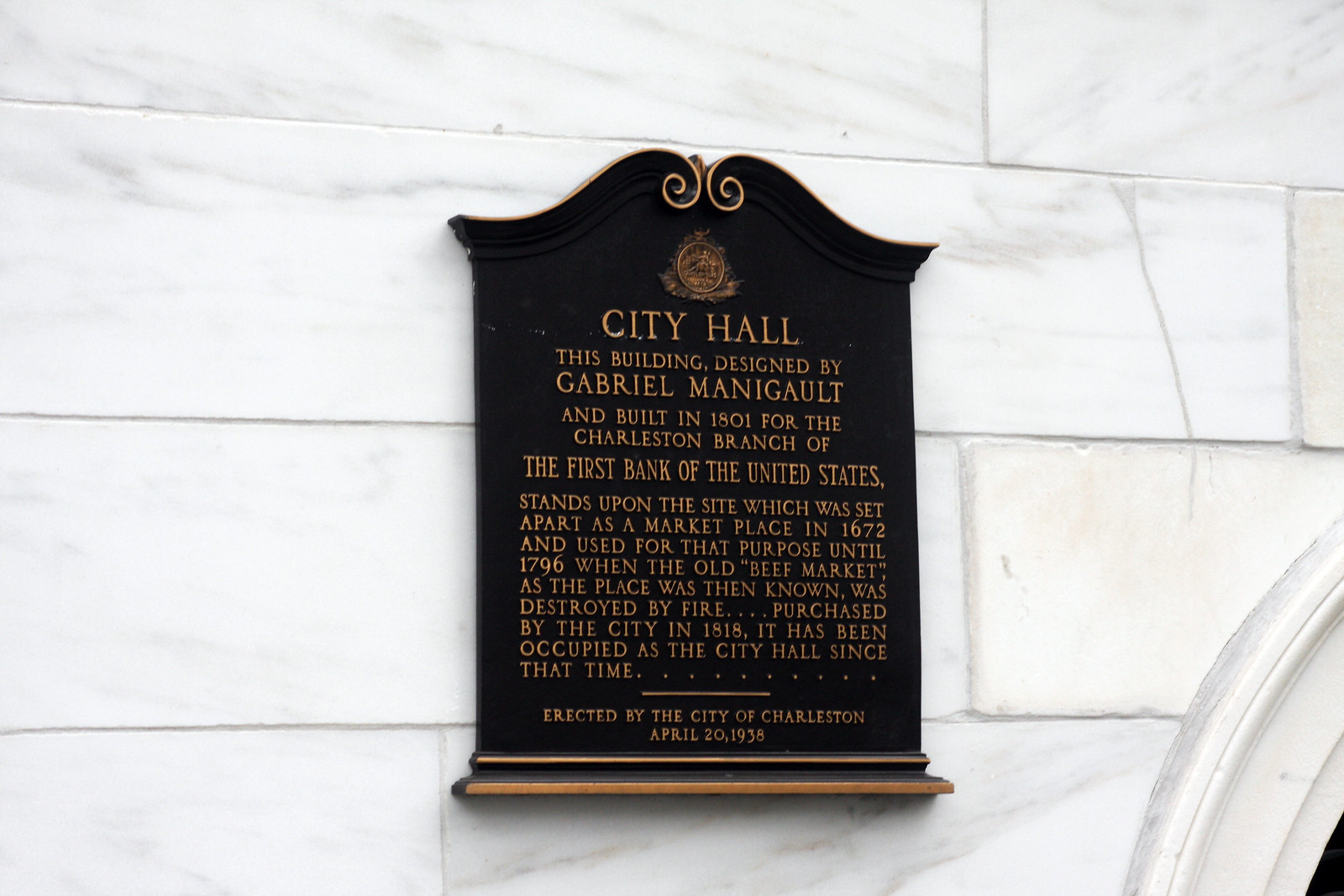In the image, a detailed and historically rich plaque is prominently displayed, affixed to a marble wall of a grandiose white brick building, known as Charleston City Hall. The plaque itself features a striking black backdrop with gold lettering, providing a stark and elegant contrast that makes the text stand out. The inscription reads: "City Hall. This building, designed by Gabriel Manigault and built in 1801 for the Charleston branch of the First Bank of the United States, stands upon the site which was set apart as a marketplace in 1672 and used for that purpose until 1796, when the Old Beef Market, as the place was then known, was destroyed by fire. Purchased by the city in 1818, it has been occupied as the City Hall since that time. Erected by the city of Charleston, April 20, 1958."

Positioned centrally in the frame, the plaque is meticulously crafted, underscoring its historical significance and the architectural beauty of the building it adorns. A nearby doorway is visible at the lower right, suggesting the image was taken outdoors, under daylight. The setting and the aesthetic elements of the image, including the use of colors like white, black, yellow, and gold, augment the grandeur and historical ambiance of Charleston City Hall.